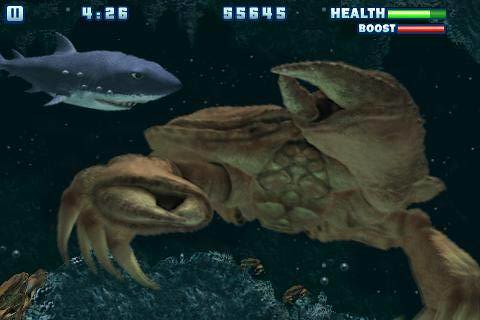In this captivating screen grab from an animated video game, we see a colossal crab dominating the underwater scene. The crab boasts impressively large claws and is cloaked in a dark reddish-tannish brown hue. To the left and slightly above the crab, a smaller but equally striking great white shark swims by, characterized by its dark gray upper body and contrasting white underside. The crab, dwarfing the shark, stands on a rock formation that resembles coral, tinged with a bluish hue, adding to the underwater ambiance. The background sets a mysterious tone, cloaked in darkness, suggesting a profound ocean depth where sunlight scarcely penetrates. Overlaying the scene, a game interface displays essential elements such as a timer, health bar, and score, adding context to the intense underwater adventure.